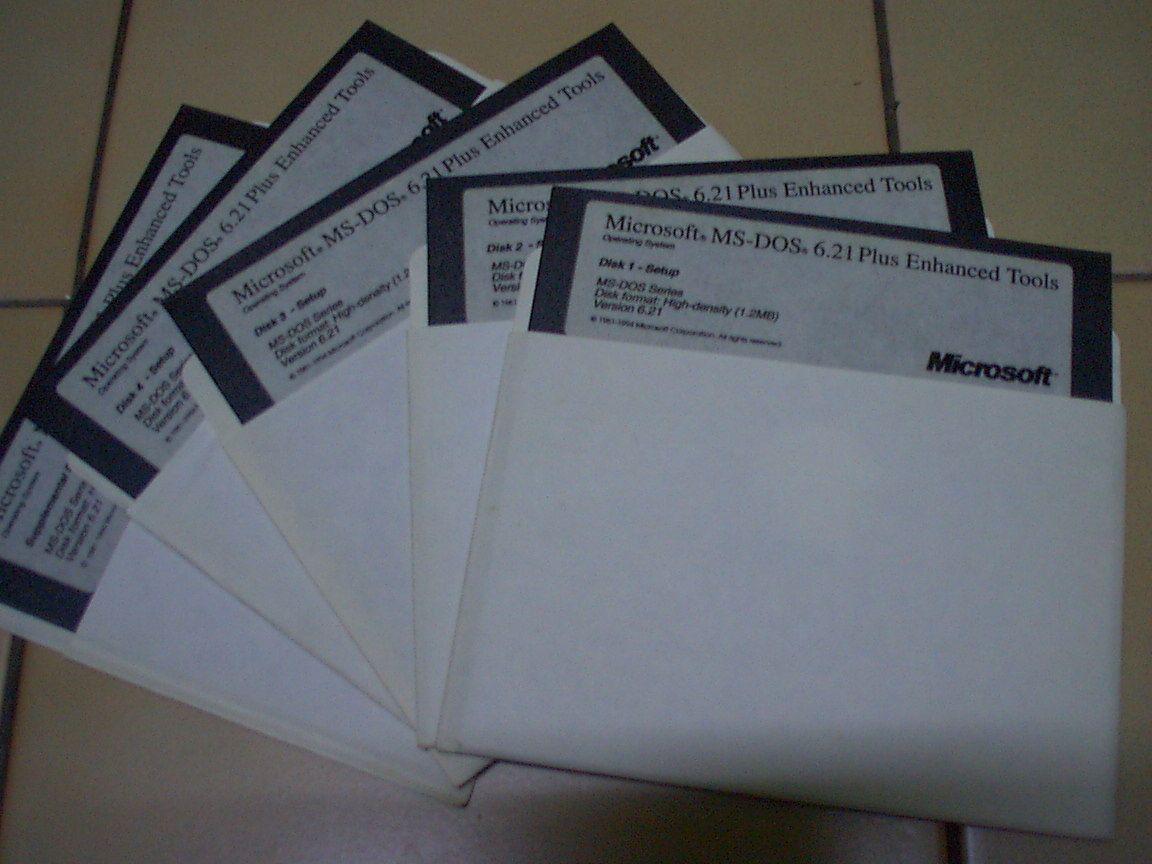This image showcases five vintage 5.25-inch floppy disks, fanned out on a light beige tile floor with dark grout. Each disk is encased in a white paper sleeve, revealing only their labels at the top. The labels, featuring a black border and white background, prominently display "Microsoft MS-DOS 6.21 Plus Enhanced Tools." Additional details include "Disk 1 Setup MS-DOS Series Disk Format High Density 1.2 Megabyte Version 6.21" and the Microsoft logo in the lower right corner. Small print with likely copyright information is also visible, though too tiny to read clearly. The disks are neatly arranged, providing a nostalgic glimpse into early computer software media.